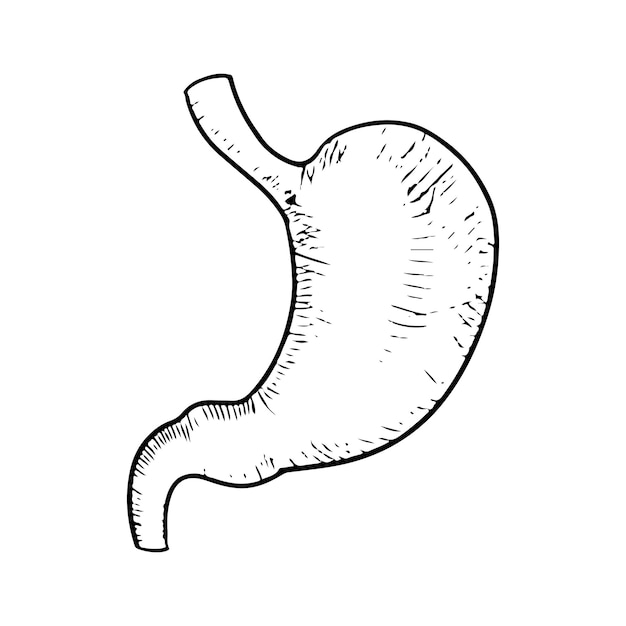The image depicts a very simplistic, black-and-white line art drawing of an anatomical stomach. It features a kidney bean-like shape with minimal detailing. The drawing is reminiscent of linoleum cutting or a stamped image, with internal lines appearing somewhat broken, possibly suggesting a well-worn or frequently copied illustration, like one that has been Xeroxed multiple times. The organ is front-facing and uncolored, showcasing only the black ink against a white background, akin to a sketch found in a medical textbook or sketchbook.